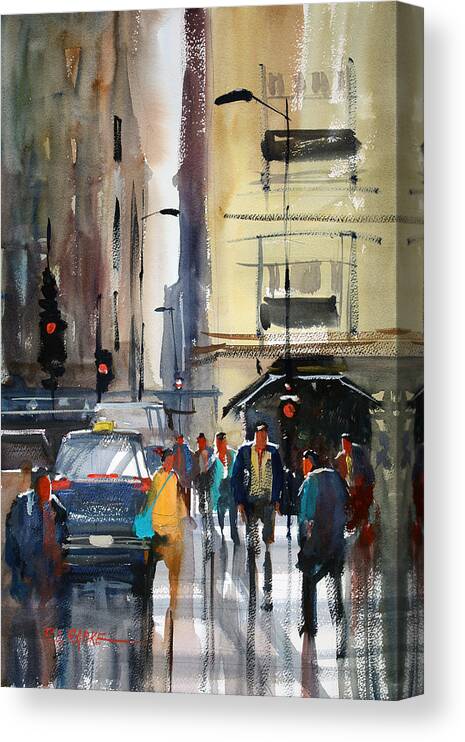This is a detailed watercolor painting in portrait mode, designed to be a 3D canvas wrap without a frame, depicting a bustling city scene. In the foreground, several people, mostly wearing business attire in shades of blue, dark blue, and tan, walk across the street and along the sidewalks, creating a sense of busyness. The atmosphere suggests it might be raining, as indicated by the dark hues and the indistinct, blurry faces of the people. A distinctive blue taxi with white and yellow accents is visible on the left side of the scene, halted at a red traffic light along with three other red traffic lights scattered throughout. In the background, a large tan and dark-colored office building looms, partially captured in the top left corner. The top right corner shows the side of the canvas with varying shades from light brown to white, resembling a cloudy skyline. The artwork is signed by the artist in red at the bottom left corner with an inscription ending in "RKE" followed by a long red stripe.